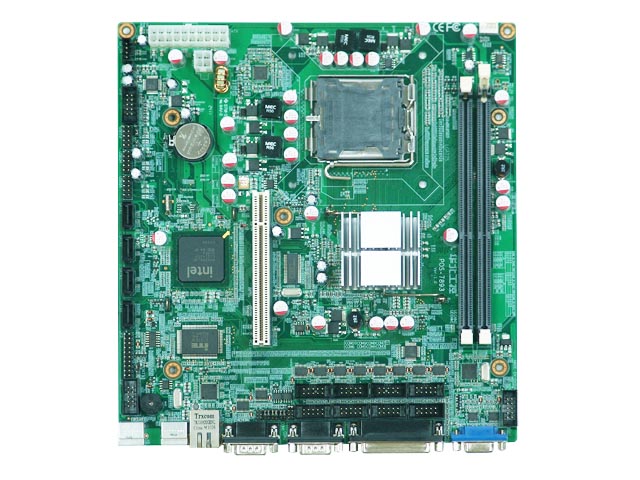This square, full-color image depicts a detailed view of a computer motherboard, primarily showcasing shades of green and silver, with accents of black and gold. At the center-left, a charcoal-colored square chip, identifiable as Intel despite being upside down, draws attention. In the upper middle section, a larger square component with a similar charcoal hue but no inscriptions is surrounded by intricate silver wires. Just above the Intel chip, there's a white rectangle with about two dozen small squares, likely a grid of connectors or circuits. Below this rectangle is a smaller white square with four square segments inside. In the upper left corner, a small silver button battery is noticeable, positioned next to a gold-colored cylinder with an open end. On the right side of the board, two long, black strips run vertically, contributing to the densely packed array of chips, circuits, and electronic components that compose this intricate motherboard layout.